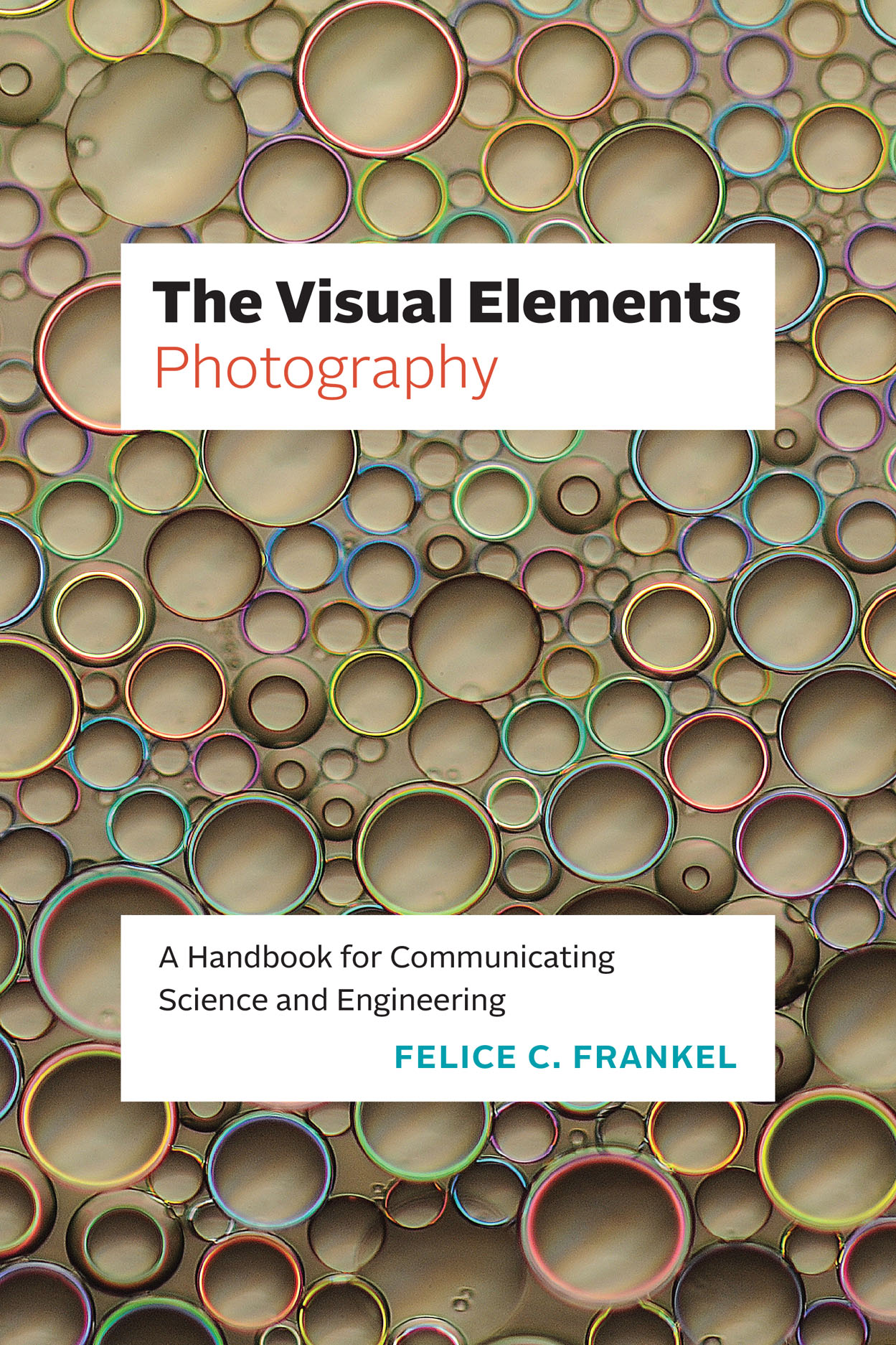This image showcases the cover of a book set against a tan background. The cover prominently features interconnected circles of various sizes, resembling colorful rings or bubbles, which create a textured, almost honeycomb-like pattern across the page. These circles come in several colors, including blue, green, pink, purple, yellow, turquoise, and gold. At the top of the cover, in bold black font, is the title "The Visual Elements," with "Photography" written just below it in orange font. Underneath these, in black font, is the subtitle "A Handbook for Communicating Science and Engineering," followed by the author's name, Felice C. Frankel, in green font. All the text is set against a rectangular white background that contrasts against the tan and colorful rings, adding a clean, structured look to the visually rich and vibrant cover.